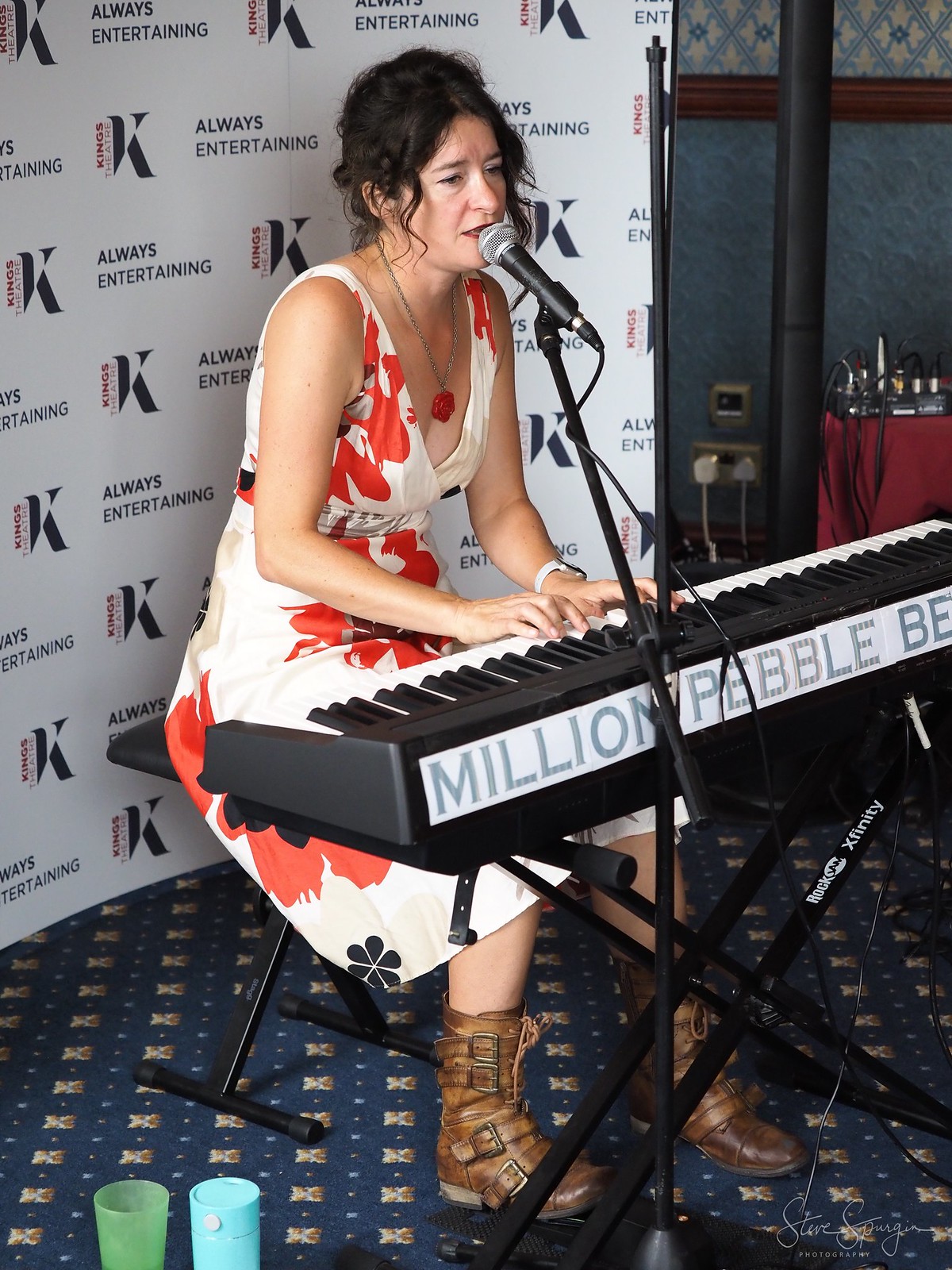In this image, a Caucasian woman with black hair, partially tucked behind her ears and back, is seated on a black stool. She's wearing a sleeveless dress with a white and orange pattern, complemented by brown boots. Around her neck, she sports a necklace with a red emblem. Her hands rest on a black keyboard, positioned on a black stand, with the keyboard’s white background displaying the text "million pebble B E." The woman is singing into a microphone attached to a stand in front of her.

Behind her, a large whiteboard prominently displays the phrase "Always Entertaining" along with a capital letter "K" that spans the board. The performance setting appears to be an indoor concert venue, as evidenced by a stage carpeted in blue, adorned with cat images and blue dots, providing an artistic touch.

In the bottom left corner of the image, there are two cups - one green and one blue. On the upper right side, a round table covered with a red tablecloth holds some black objects. Additional background details include a dark wall, a black pillar, and visible switchboards with plugged-in extension cords and equipment. All of these elements contribute to a rich and vivid scene of a musical performance.